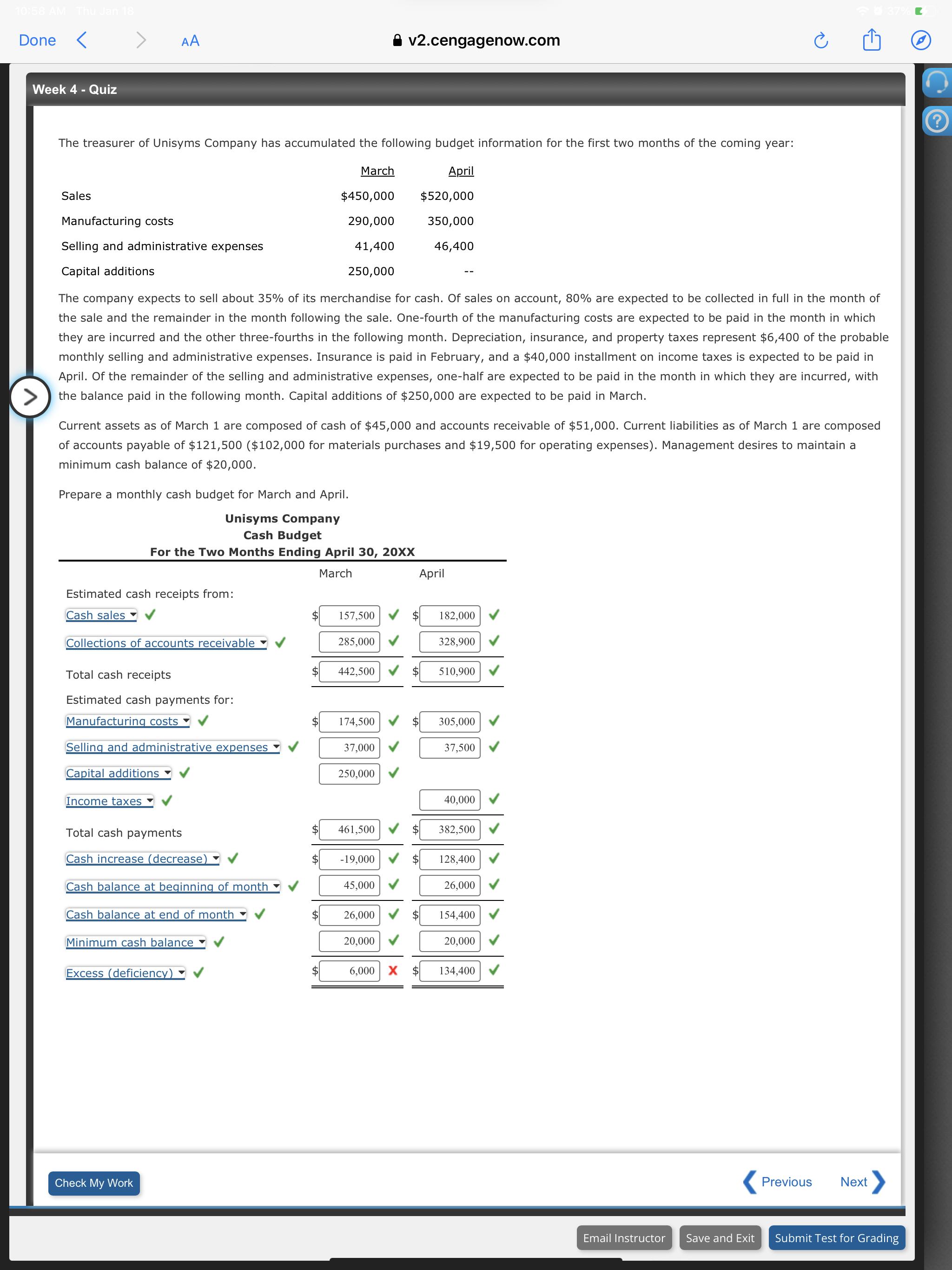The image depicts a detailed web page. At the very top, there's a light gray banner featuring the text "Done" in blueprint color, with a capital 'D'. Directly below this, a blue arrow points to the left and a gray arrow points to the right. Two capital 'A's are also present, with one being smaller and the other larger, possibly indicating text adjustment options.

In the center of the page, there's a padlock icon accompanied by the text "V2.cengagenow.com," suggesting a secure connection to the website. To the right, icons for upload and refresh functions are displayed.

A wider black banner extends from the center, bordered by a gray line, dominating most of the page. This banner contains the title "Week 4 - Quiz" and a subheading "The Treasurer." The background here is gray, contrasting with the text inside.

The document outlines budget information for Unisim's company for the first two months of the forthcoming year under various categories:
- Sales: $430,000 in March and $520,000 in April.
- Manufacturing Costs: $290,000 in March and $350,000 in April.
- Selling and Administrative Expenses: $41,400 in March and $46,400 in April. 
- Capital Additions: $250,000 in March, with April left blank.

Further details continue with an explanation about the company and the cash budget summary for the two months ending April, quantified as $32,000 XX. The text continues to break down the estimated cash receipts, total cash receipts, estimated cash payments, and total cash payments, providing comprehensive financial information.